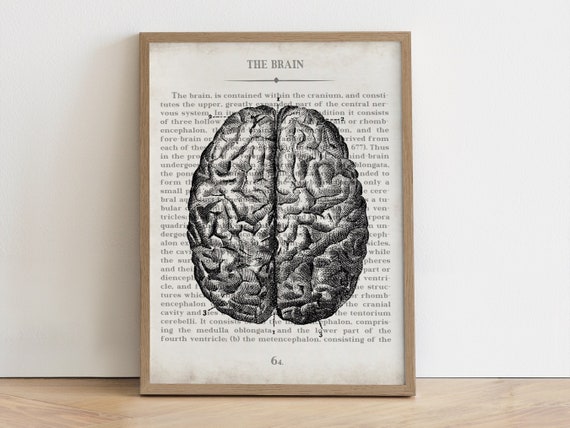The image depicts a photograph of an old, weathered textbook page framed and displayed as a piece of art. The framed page leans against a white wall on a natural hardwood floor. The frame is thin and wooden, giving it a rustic feel. The page, appearing slightly browned with age, is from a science or medical textbook and prominently features the heading "The Brain" in capital letters at the top. Below the heading is a realistic, black-and-white illustration of a brain, intricately detailed with all its curves and sections, likely rendered in charcoal or pencil. 

The illustration is overlaid on descriptive text that delves into the anatomy of the brain, starting with "The brain is contained within the cranium and constitutes the upper, greatly expanded part of the central nervous system." Although some portions of the text, especially over the darker areas of the brain illustration, are difficult to read, it mentions the brain's structural components such as the medulla oblongata and the rhombencephalon. A horizontal line separates the heading from the main body of text. Notably, the bottom of the page is marked with the number "64," indicating its original place in the textbook.